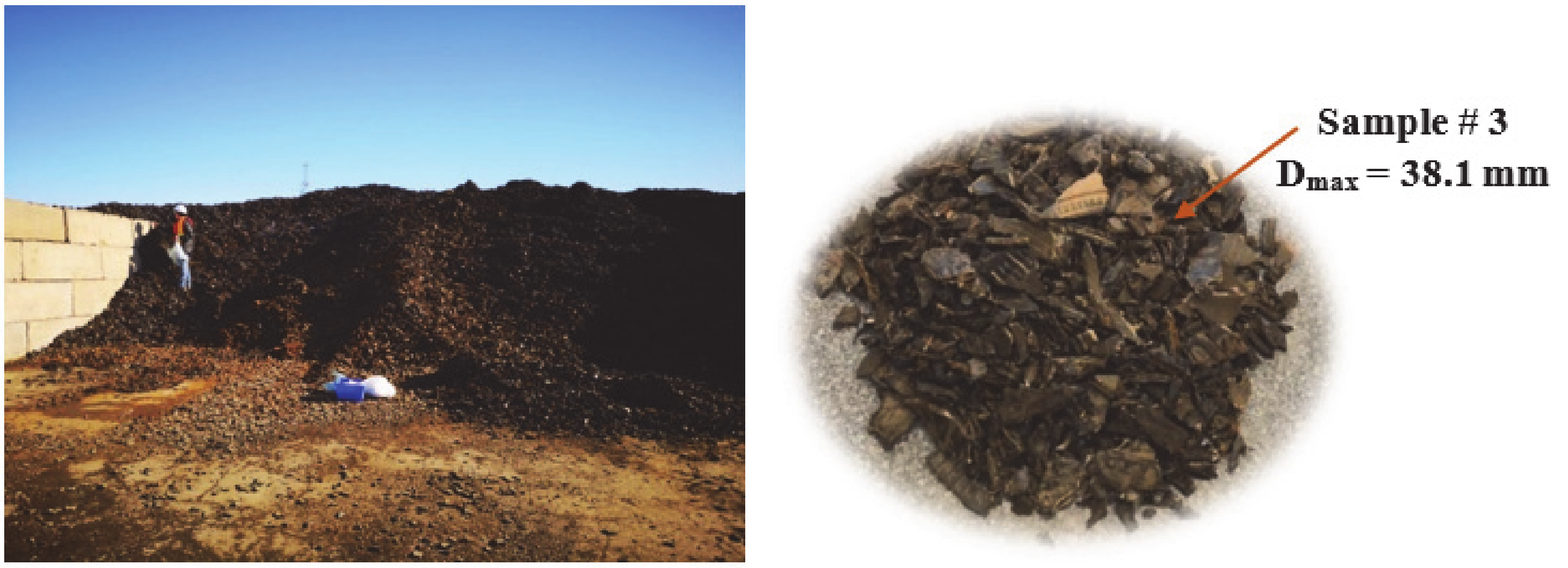The image consists of two side-by-side pictures. The left photograph depicts an outdoor area where a man, wearing a white hat and an orange high-visibility vest, is climbing a minor hill made of dark brown gravel-like debris. A plastic bucket and a white bag are visible at the base of the mound. Cinder blocks form a makeshift wall on the left side of the image. The sky is clear and blue. The right image is a close-up of the same dark debris, showing random shapes placed in a circular manner. An orange arrow points towards the debris with black text that reads, "sample hash 3D max = 38.1 mm," on a white background.